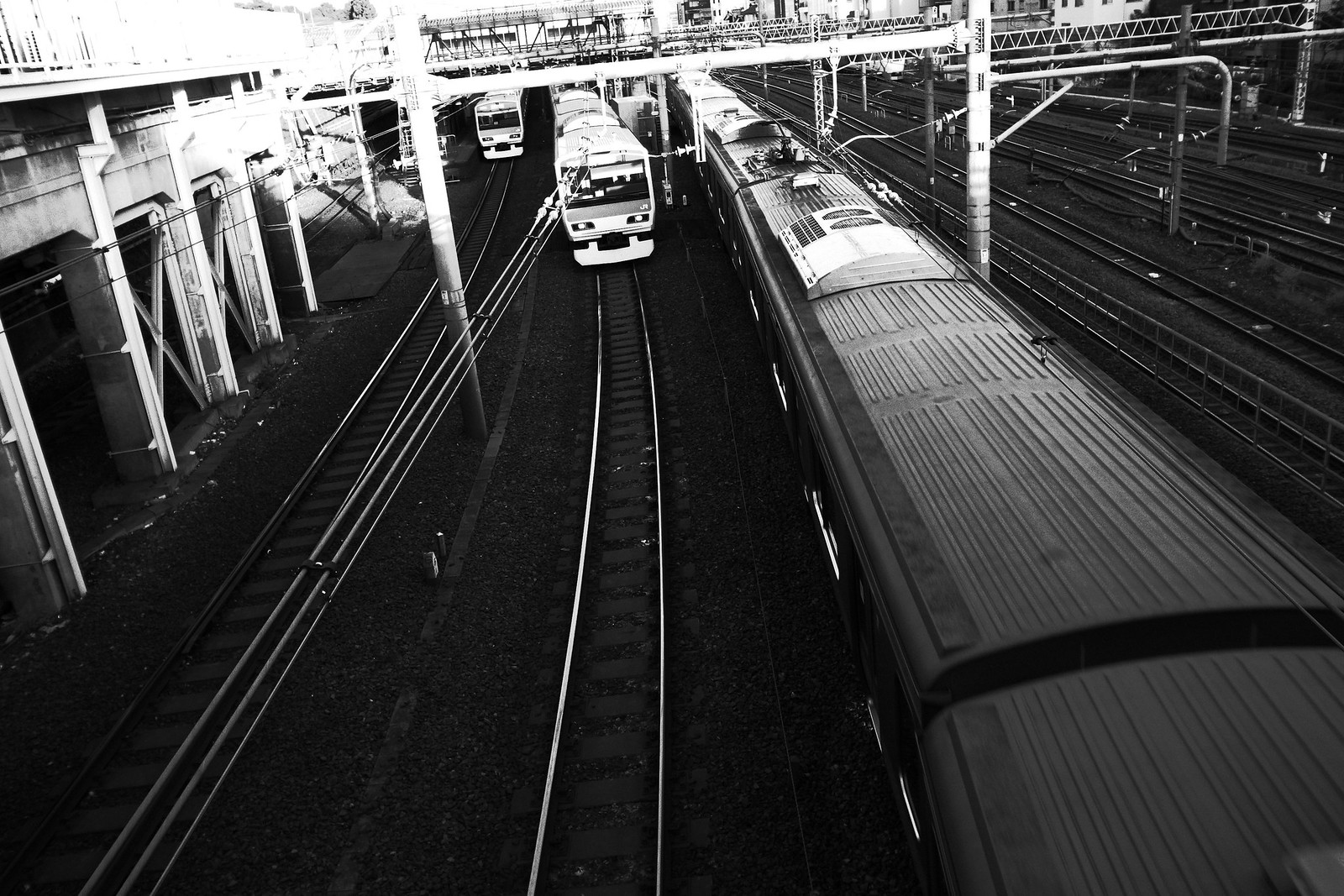In this black and white photograph, we see an industrial railway station bustling with activity. The image captures multiple train tracks, specifically highlighting the six most prominent ones. On the three leftmost rails, there is an array of trains. The rightmost train among these three occupies the entire length of its track and is positioned nearest to the viewer. Moving left, a second train can be seen approaching the foreground, distinctive with its white exterior and a noticeable brown stripe along its front. Further back on the leftmost track, another white train with a brown front line is slightly behind the second train, also moving towards the camera. 

The tracks not occupied by trains remain empty, emphasizing the active yet orderly nature of this station. Surrounding the scene are white metal columns supporting overhead spans, possibly a bridge or overhead structure, ensuring safety and adding to the industrial atmosphere. Steel beams crisscross the upper portion of the image, adding to the structural integrity of the area. The photograph, framed by these elements, vividly conveys a sense of relentless motion and the practical, robust design typical of a busy railway hub.